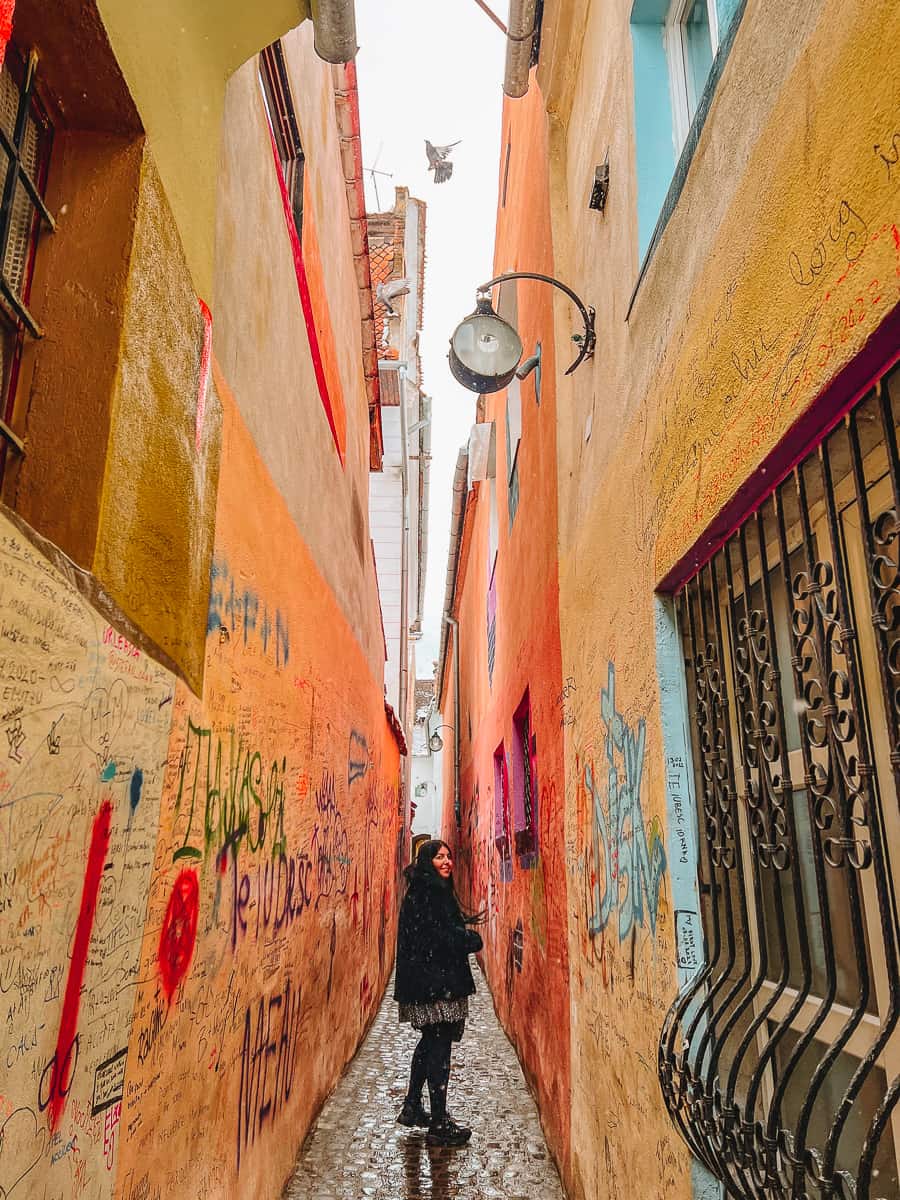In the image, a young woman with dark hair, dressed in a black coat, a black and white skirt, black leggings, and black shoes, walks through a narrow alleyway between two buildings. The cobblestone path she treads is distinctly narrow, to the extent that she could easily touch each building if she stretched out her arms while standing in the middle. The buildings, two stories tall and adorned in shades of orange, tan, beige, peach, and light blue, are heavily graffitied, with names and art splashed across the walls, suggesting frequent use by passersby commemorating their journeys.

She looks back over her shoulder, smiling warmly at the camera. Intricately wrought ironwork and simpler grates cover the building’s windows, specifically a notable decorative grate on the right side of the photo. Above, lights are attached throughout the pathway, ensuring the alleyway is well-lit at night. A bird is caught in mid-flight in the narrow gap at the top of the buildings, heading upwards and to the left. Snow is gently falling, the flakes more discernible against her black coat. Additionally, a peculiar metal object hangs off one of the buildings, featuring a half-circle and a circular white center, adding an enigmatic charm to the scene.